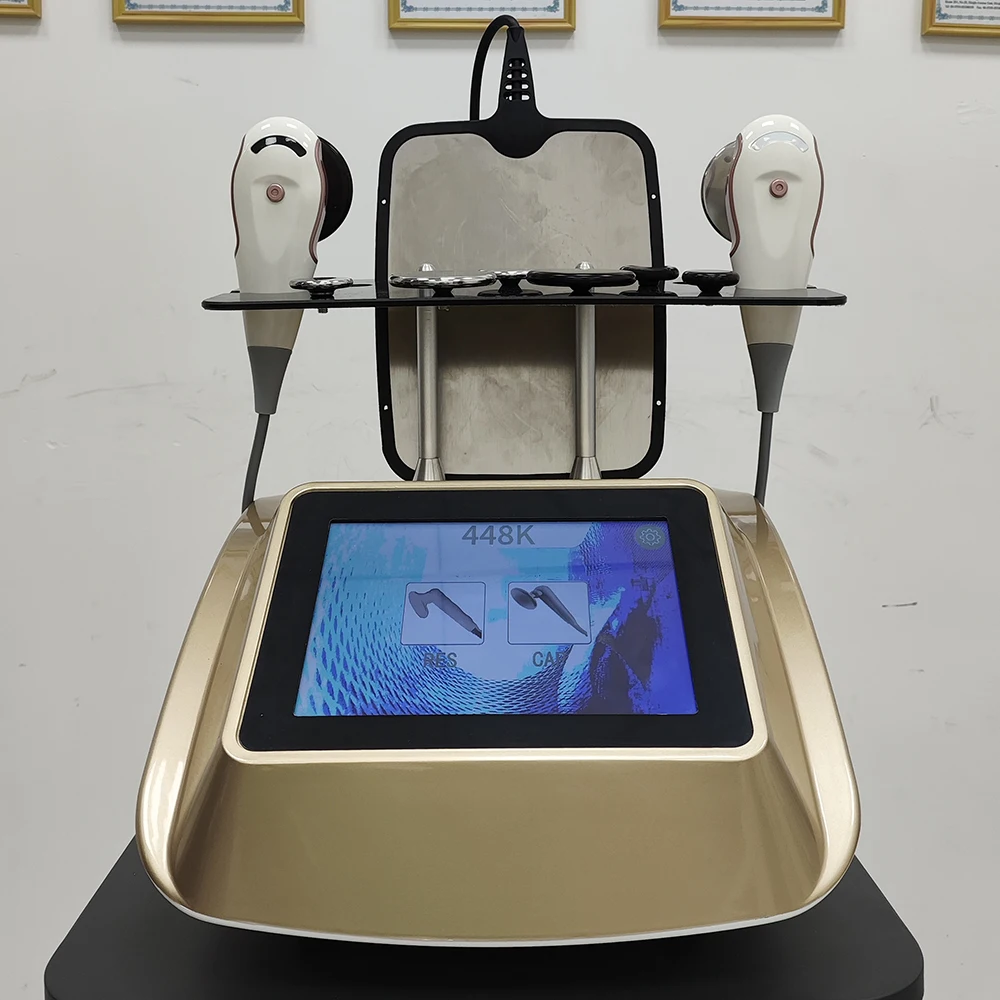This indoor photograph appears to be taken in a medical office or clinical setting. The main focus of the image is a black desk or tabletop that supports a large, brass-colored base, which houses an LED screen displaying '448K' against a blue background. The screen includes images of two teardrop-shaped paddles or wands, which are labeled 'Rez' on the left and 'Cap' on the right. Above this, resting within a black case, is a larger vertical object with a flat panel, also connected by a black cable. Flanking this object are two white, teardrop-shaped devices connected by gray cables, possibly resembling ultrasound wands. The background features a white wall with subtle scratch marks and a row of gold-framed certificates or plaques at the top, suggesting a formal medical environment.